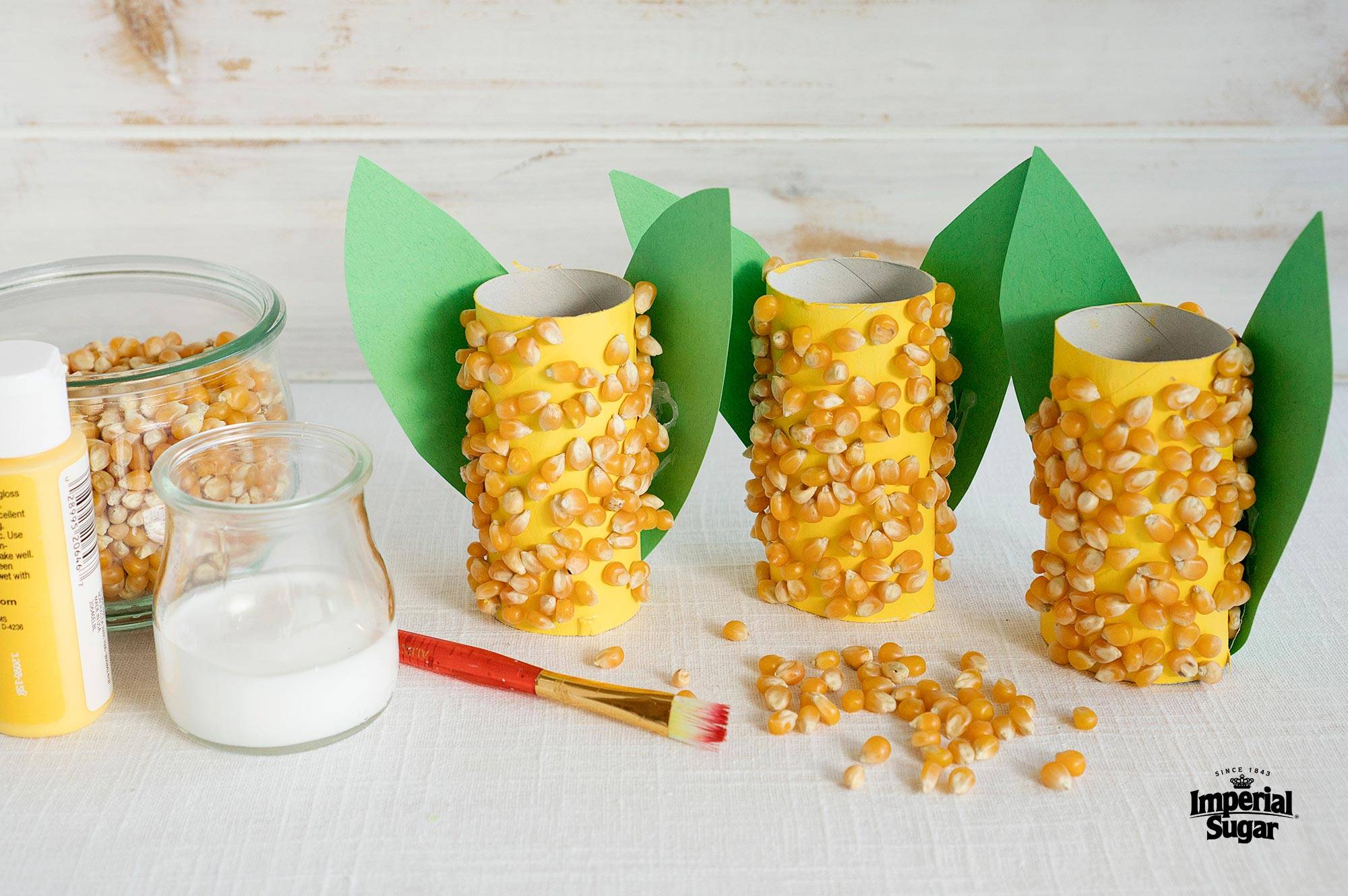This photograph captures a detailed scene of a children's arts and crafts project. The centerpiece consists of three hollow cylinders, likely reclaimed toilet paper rolls, each wrapped meticulously in yellow construction paper and adorned with glued popcorn kernels. Large, green crepe paper leaves are affixed to the back of each cylinder, two per roll, making a total of six leaves. These artistic elements are arrayed on a stark white surface.

In the foreground, additional loose corn kernels are scattered, contributing to the tactile quality of the project. Also prominent are a red paintbrush and a small glass container, potentially used for dispensing the adhesive that affixed the kernels; this container holds a white substance that could be either paste or glue. To the left, a yellow bottle with a white cap, possibly containing more glue or paint, stands beside a glass bowl nearly filled with corn kernels.

The background is made up of horizontal white planks, adding to the clean aesthetic of the scene. A faintly stained white countertop supports the entire arrangement. In the lower right-hand corner of the image, the "Imperial Sugar" logo is visible, subtly branding the photograph.